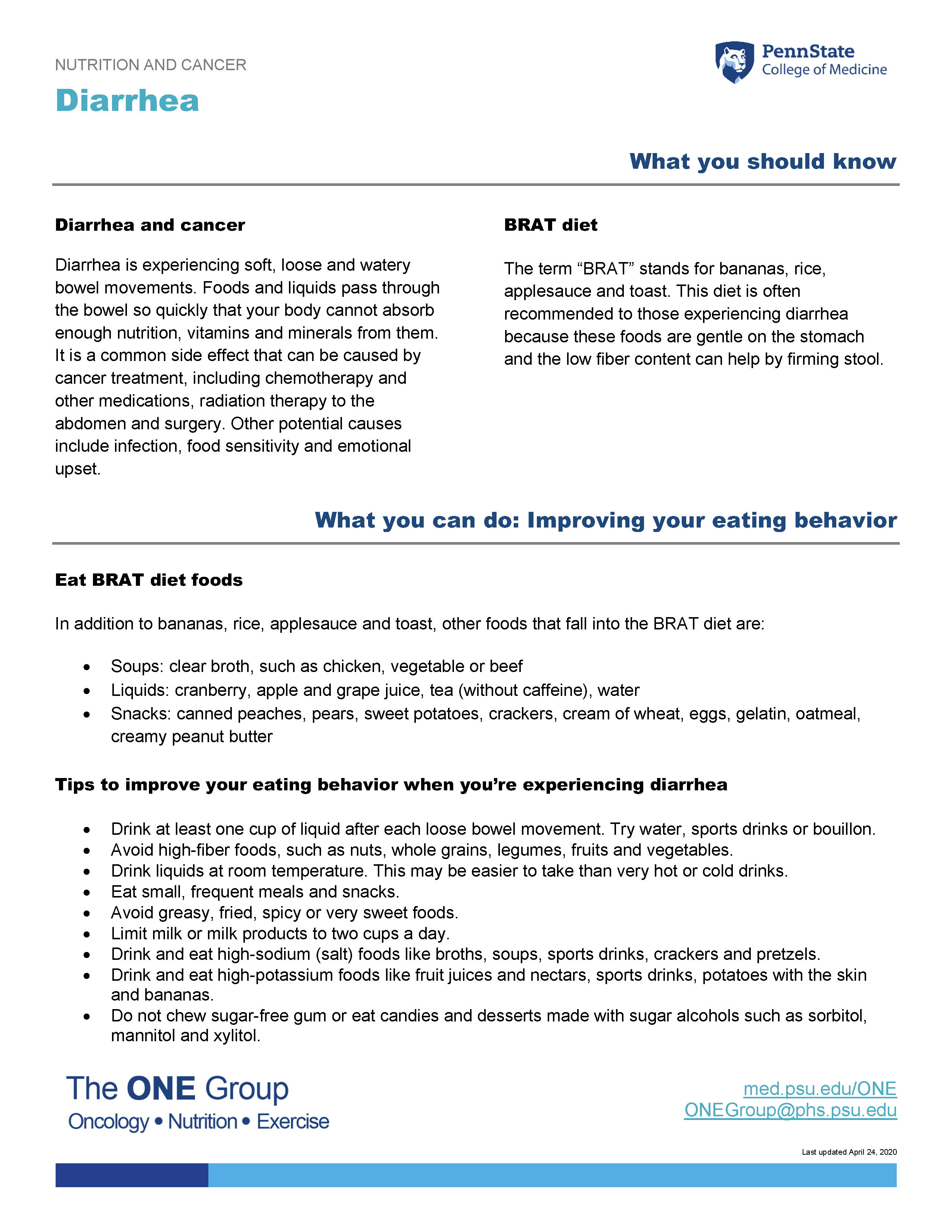The image depicts an 11x14 printed medical information page with a white background. At the top left in black text, it reads "Nutrition and Cancer," followed by "Diarrhea" in light blue. On the upper right, there is a Penn State College of Medicine logo featuring a lion's head within a blue shield, and beside the logo reads "Penn State College of Medicine" and "What You Should Know" in dark blue. A black horizontal line separates the header from the contents below.

The main content is structured into two columns of text and several sections with various headers in dark and light blue. The top left section titled "Diarrhea and Cancer" describes the condition as involving soft, loose, and watery bowel movements that impede nutrient absorption, often as a side effect of cancer treatments such as chemotherapy, radiation therapy, and surgeries. Below it, headings provide further details, such as specifying other potential causes like infections, food sensitivities, and emotional distress.

In the top right section, bolded text introduces the "BRAT diet," explaining that the acronym stands for Bananas, Rice, Applesauce, and Toast, which are gentle on the stomach and can help firm stools. Detailed bullet points list recommended foods and drinks, including clear broths, certain juices, tea without caffeine, gelatin, and more.

Further down in these sections, under a blue header reading "What You Can Do, Improving Your Eating Behavior," the document elaborates on actions to take, advising to "Eat BRAT Diet Foods" and offering numerous bullet-pointed recommendations. These include drinking a cup of liquid after each loose bowel movement, avoiding high-fiber foods, eating small frequent meals, and limiting high-fat, spicy, and very sweet foods. It also suggests focusing on high-sodium and high-potassium foods and avoiding sugar-free gums and candies with sugar alcohols.

At the bottom left, the document is signed off with "The One Group Oncology Nutrition Exercise" in blue text, and to the right, in lighter blue, it includes the web address "med.psu.edu/one" and the email "onegroup@phs.psu.edu." There is a navy blue and light blue banner at the bottom, visually enclosing the footer information.